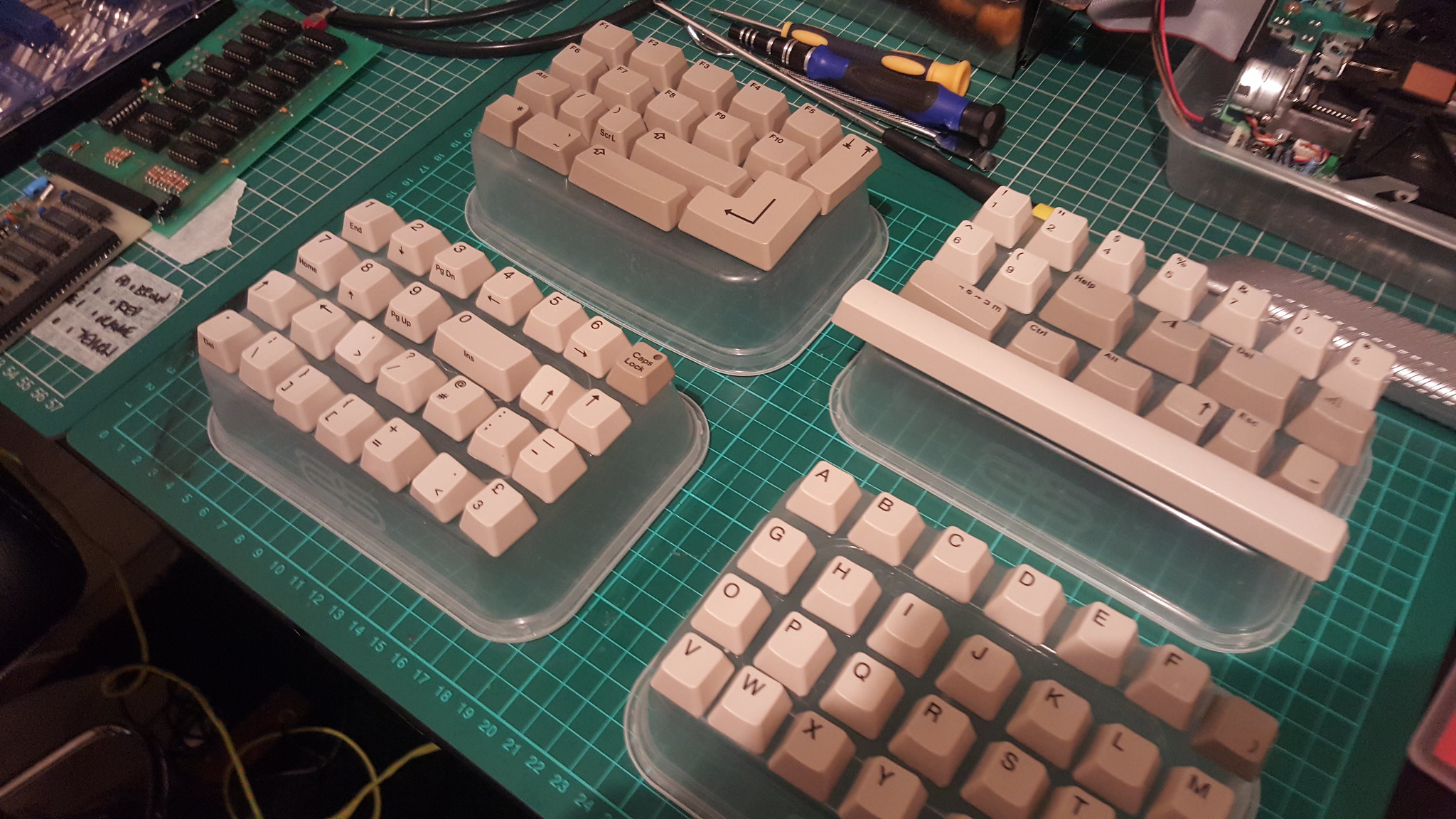The image showcases an organized workspace, likely a mechanical workshop. The focal point is a table covered with green graph paper, featuring a grid with numbered axes ranging from 0 to 24. This setup appears to be used for precise measurements. The table holds an array of mechanical keyboard components, each positioned on overturned Tupperware containers. The keycaps vary in color: beige, white and beige, and white with black lettering. Surrounding the keyboards are various electronics, including motherboards and circuit boards. Detailed circuit boards lie to the left, some with labels and small rivets visible. The workspace also contains tools such as screwdrivers and scattered wires on the floor below, contributing to an atmosphere of active tinkering and assembly.